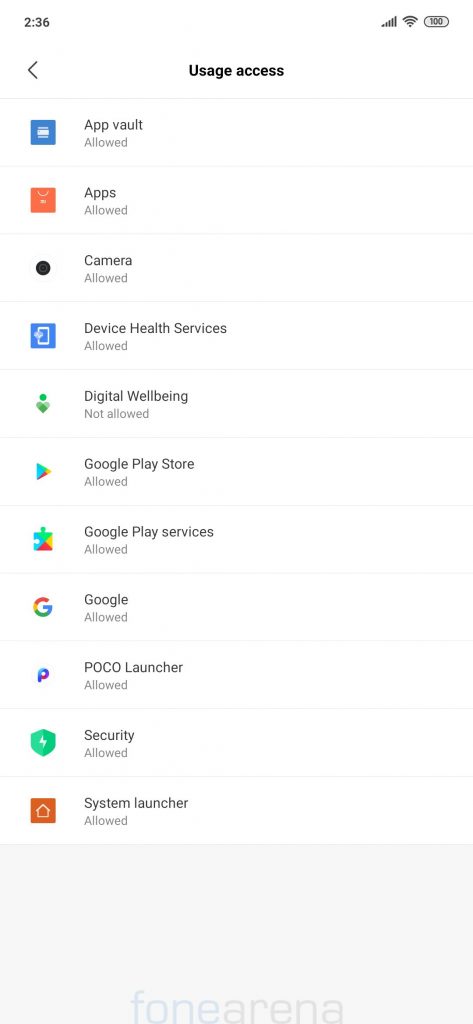This screenshot captures the Usage Access settings page on a smartphone with a white background. The time is displayed as 2:36 in the top left corner, while icons for battery, Wi-Fi, and signal strength are situated in the top right corner. The title "Usage Access" is centrally positioned in black text at the top of the page, with a left-facing caret icon aligned on the same horizontal plane to its left.

Below this header, there is a detailed list of apps, each accompanied by its respective icon on the left. The names of the apps are written in black text, followed by a status in gray text beneath each name indicating whether access is "Allowed" or "Not allowed." Specifically, the list includes:
- App Vault (Allowed)
- Apps (Allowed)
- Camera (Allowed)
- Device Health Services (Allowed)
- Digital Wellbeing (Not allowed)
- Google Play Store (Allowed)
- Google Play Services (Allowed)
- Google (Allowed)
- POCO Launcher (Allowed)
- Security (Allowed)
- System Launcher (Allowed)